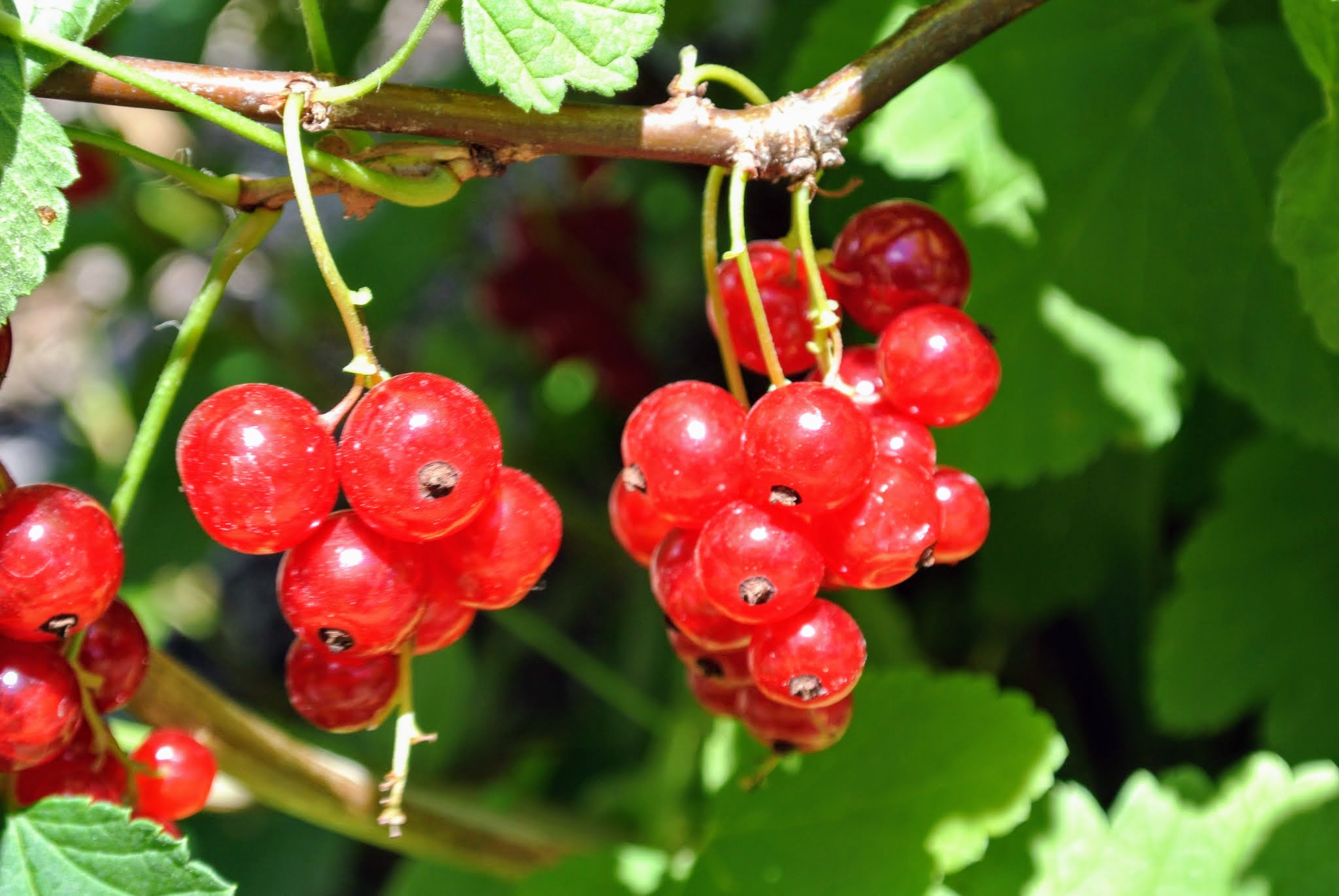This is an outdoor, close-up photograph of red, round, shiny berries growing in clusters on thin green stems. The primary focus is on approximately five clusters, each containing about three to five berries, arrayed across the shot. The stems extend from a brown branch that loops down from the top of the image. The clusters are strategically positioned, with the largest group located center-right and including one larger berry in the shade. Surrounding the berries, there are slightly smaller leaves growing off the stems, with larger fan-like green leaves creating a blurred, sunlit background. The overall scene captures the vibrancy and texture of the berries and the greenery in vivid detail.